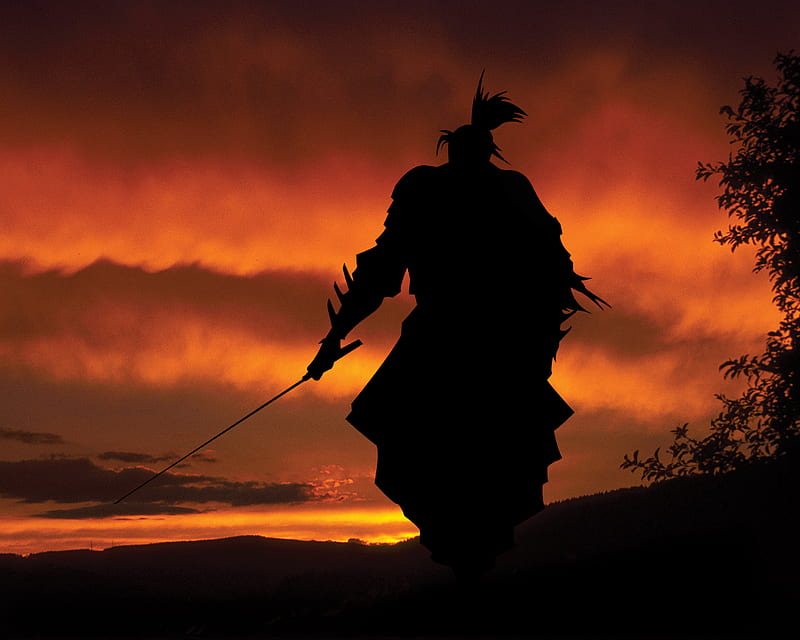In this dramatic image, we see the black silhouette of a samurai standing prominently in the foreground. The samurai, adorned in intricate armor complete with wrist guards that have menacing spikes, stands on a hill with a large, thin-bladed katana held in his right hand. His hair is tied back in a distinctive ponytail. The background is an intense spectacle of red and dark orange hues, depicting a fiery sunset partially obscured by large clouds. To the right of the image, there is a tree with serrated leaves, its form also cast in deep shadow. The samurai gazes towards the horizon, where a series of rolling hills can be faintly discerned beneath the rich, glowing sky, enhancing the mystique and solitude of the scene. The overall aesthetic of the image resembles a stylized animation, adding to its strikingly cinematic quality.